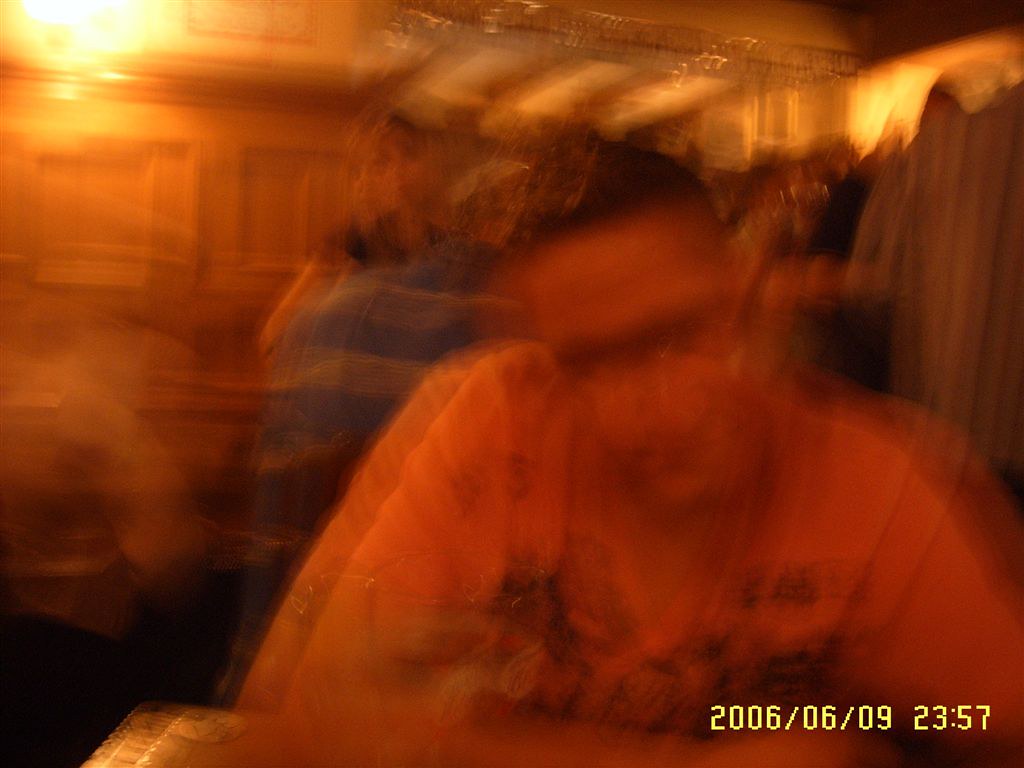The blurry, dark-colored photograph from June 9, 2006, timestamped at 23:57, appears to capture a scene in a restaurant or similar interior space. Dominating the bottom right corner of the image is a man with short dark hair and dark eyebrows, wearing a peach-colored V-neck shirt with an indistinguishable design. He sits at a table with his arms crossed, leaning slightly forward and tilting his head to the left as he looks towards the camera. The dim lighting suggests a darker atmosphere, accentuated by a prominent light shining down from the upper left-hand corner. In the background, a woman with dark hair and a horizontal striped shirt—dark blue and light blue or gray—stands, possibly holding something. The setting is characterized by a decorative wooden wall, a likely black floor, and curtains or wooden cupboards. A blurred figure can also be seen to the left, indicating movement, while the yellow digital timestamp in the bottom right corner clearly marks the date and time.